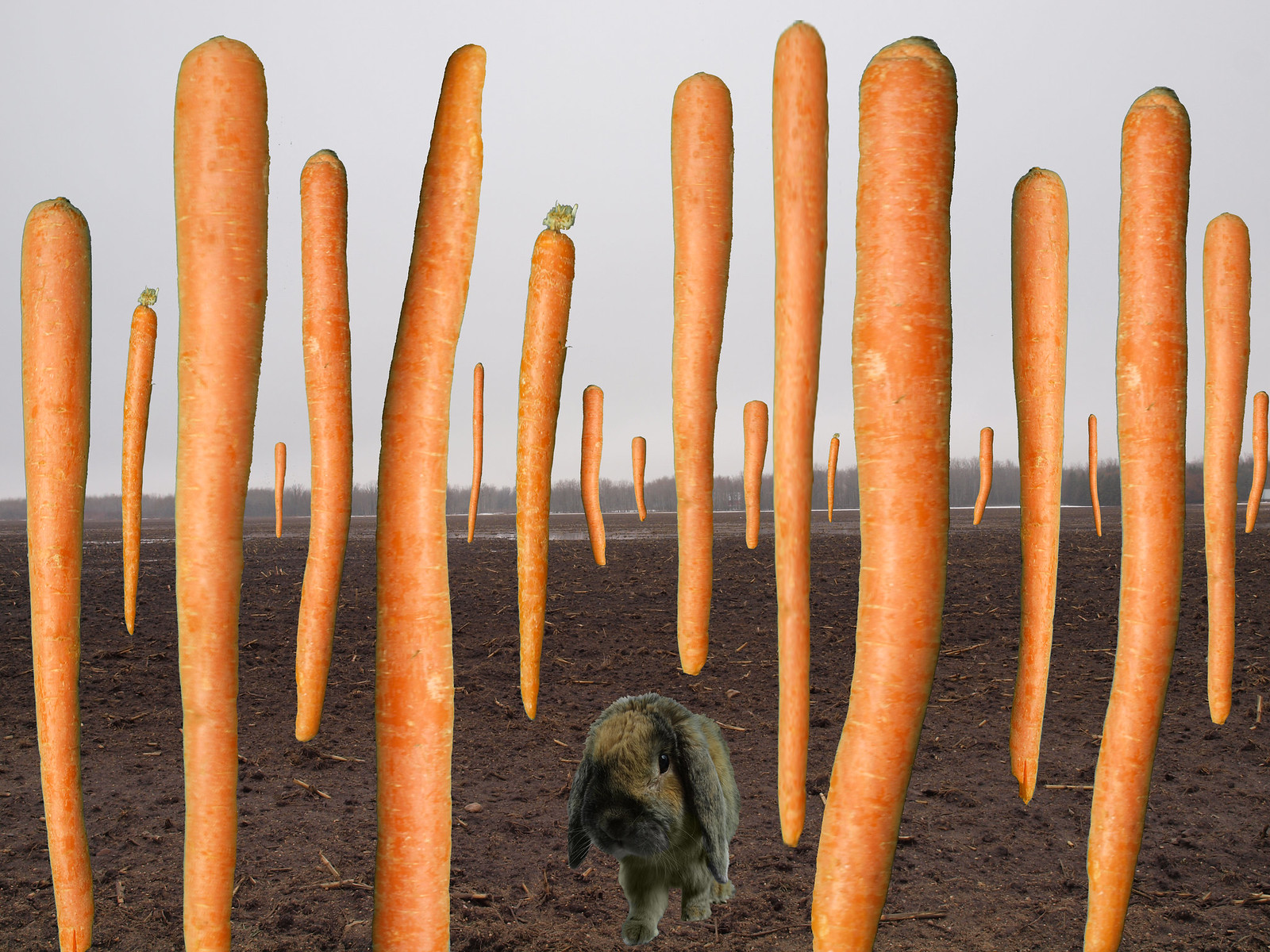In the center of this surreal, Photoshopped image, a small, brown rabbit with detailed black and gray streaks sits with its little black eyes gazing forward. The rabbit has long, floppy ears with patches of light brown and gray, and a dark muzzle with a diagonal streak of brown across its face. It rests on a brown, muddy field, littered with a few sticks. Surrounding the rabbit are excessively large, vertical carrots, some with and some without green stems, standing erect like pillars stretching into the distance. The field extends back to a tree line of bare, autumnal trees under an overcast sky that mixes shades of gray and hints of blue. The image is wider than it is tall, capturing an almost fantastical scene of repeated carrot pillars that enhance the overall surreal and photomontage-like quality of the composition.